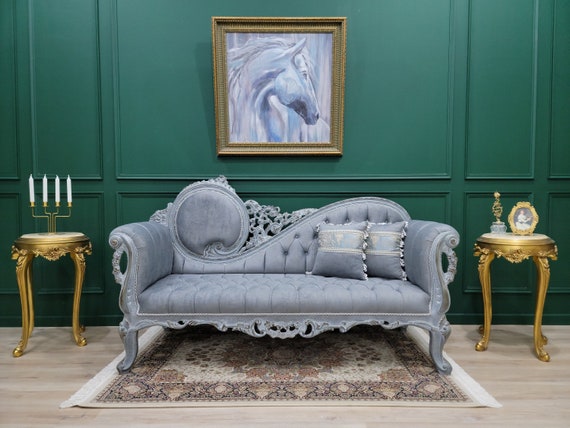The image depicts an ornate room with vivid green walls and hardwood flooring. At the center, a lavish loveseat, which appears to be upholstered in velvet, sits atop a somewhat faded tan and red rug. The loveseat features intricately curled arms, a unique rounded back that curves elegantly upward, and filigree detailing. Flanking the loveseat are two four-legged gold end tables, each topped with what seems to be marble surfaces. The table on the right holds a decorative knickknack beneath a gold-framed picture, while the one on the left supports a candle holder with four candles. Above the loveseat hangs a sophisticated watercolor painting of a horse's profile, also framed in gold. Completing the scene are throw pillows on the loveseat that complement its luxurious appearance.